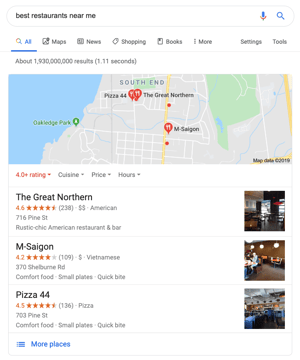The image depicts a Google search results page for "best restaurants near me." At the top, the search bar is visible alongside icons for voice input and standard search. Beneath the search bar, there are navigation tabs labeled "All," "Maps," "News," "Shopping," "Books," "More," "Settings," and "Tools." The search query yielded approximately 1.93 billion results in 1.1 seconds.

Displayed below the search details are listings of various restaurants. The first notable entry is "Pizza 44" located in The Great Northern shopping area. For each restaurant, there are clickable options for "4+ rating," "cuisine," "price," and "hours." 

The locations captured include Oak Bridge Park, Mt. Saigon, and South End, shown on a map. 

1. **Great Northern**: 
   - Address: 716 Pine Street
   - Description: Rustic chic American restaurant and bar
   - Visual: Interior photograph of the establishment

2. **Mt. Saigon**:
   - Rating: 4.2 stars from 109 reviews
   - Cuisine: Vietnamese
   - Address: 370 Shelburne Road
   - Features: Comfort food, small plates, quick bites
   - Visual: Interior scene of diners enjoying their meals

3. **Pizza 44**:
   - Rating: 4.5 stars from 136 reviews
   - Cuisine: Pizza
   - Address: 703 Pine Street
   - Features: Comfort food, small plates, quick bites
   - Visual: Photograph showcasing the restaurant's interior

Finally, there is a "More places" option highlighted in blue, encouraging users to explore additional restaurant listings.

This detailed caption encapsulates the elements present in the search results, including various restaurant details and visuals.